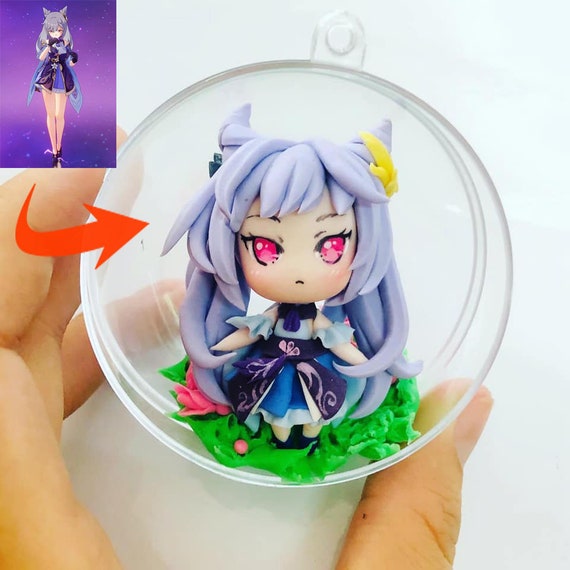The image captures a close-up of a person with medium skin tone holding a clear, round acrylic ornament with a small hook on top. Inside the ornament is a doll-like, cartoon figure of a little girl with long, lilac-colored hair tied into two horn-like ponytails, adorned with a yellow barrette on the left and a blue barrette on the right. She has striking pink eyes and a small curved down black mouth, and she wears a knee-length dress with gathered skirts in shades of blue, purple, and pink designs. The figure stands on a patch of green clay that resembles grass or leaves. The overall design gives a whimsical, anime-inspired look to the toy figure enclosed in the delicate, glass-like ornament.